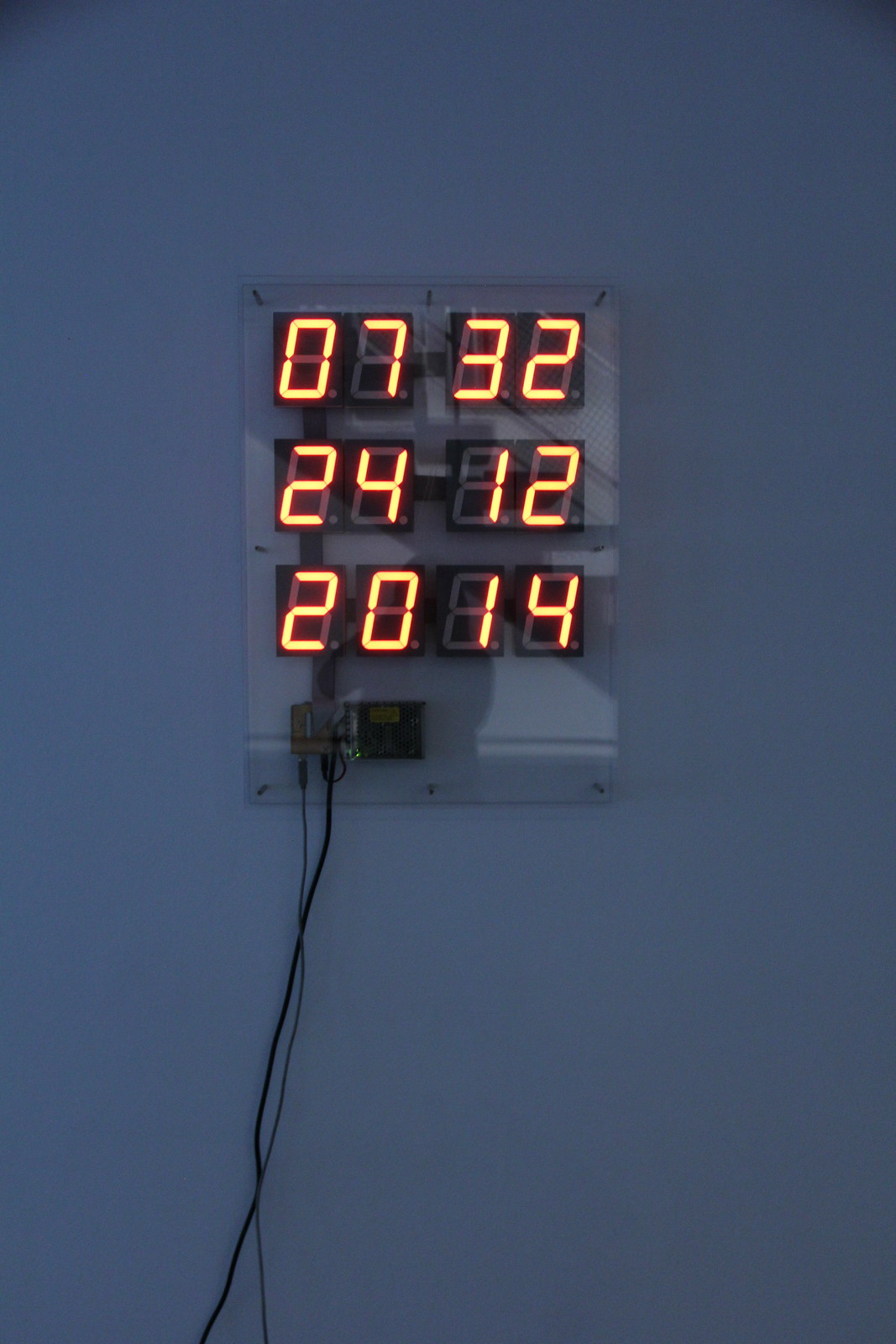The image depicts a digital sign, which is a clear rectangular display mounted against a dark navy blue background. From the bottom left of the sign, a couple of cords connect to a small black box, presumably serving as a power source for the device. The sign appears to function as a scoreboard or countdown clock, displaying numbers in three distinct rows. The top row shows "07" and "32", the middle row displays "24" and "12", and the bottom row reads "20" and "14". Each number is clearly visible against the transparent display, providing a neat and organized sequence of values.